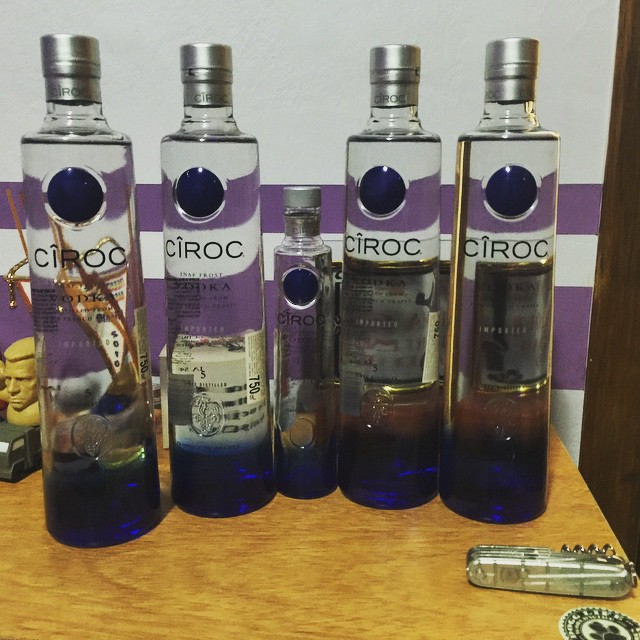The image depicts five clear glass bottles of Ciroc vodka, each marked with the brand name "C-I-R-O-C" and the word "VODKA" beneath it. Of the five bottles, four are 750 milliliters, a standard size, while the one in the center is notably smaller. Each bottle is topped with a silver lid and features a distinctive navy blue circle near the top, situated just above the brand name. The bottles also have bases tinged with blue and a faint logo, which might resemble flowers, though it's hard to distinguish clearly.

The bottles are arranged on a light brown, tan wooden table. A silver Swiss Army knife or corkscrew is also on the table, along with a small, blurry black and yellow logo sticker at the bottom. The background showcases a painted wall with alternating purple and white stripes, providing a contrasting backdrop to the glass bottles. Additionally, a partially visible man's figurine head and possibly a truck can be seen peeking out from behind the bottle on the far left.